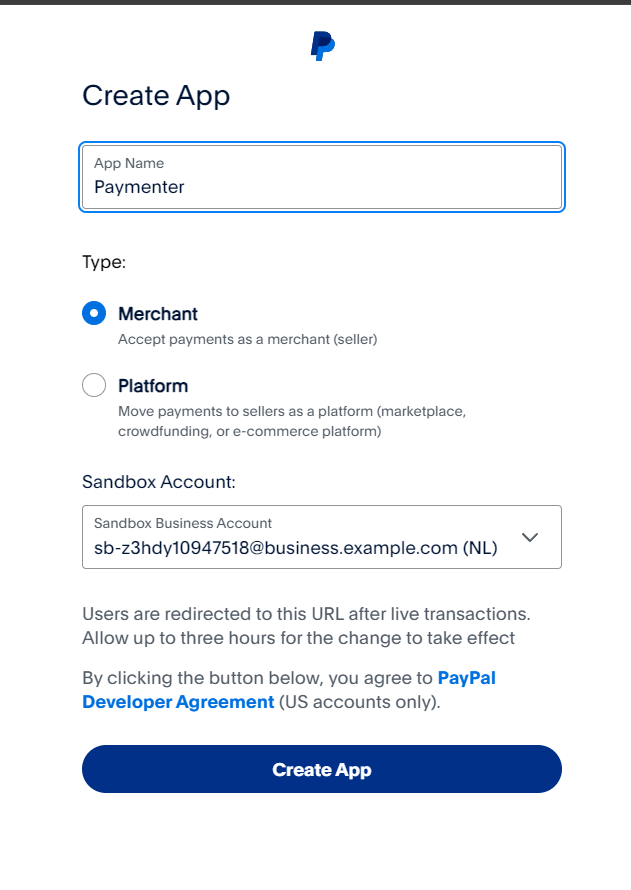In this image, we see a PayPal page dedicated to the creation of an app. At the top of the page, the PayPal logo is prominently displayed, consisting of two interlocking P's—one dark blue and the other light blue. The header text reads "Create App." Following this, the page outlines the requirements for creating an app, specifically tailored for merchants and platforms. 

The app is named "Paymenter" with the type specified as "Merchant." This designation allows the app to facilitate payments for merchants and sellers on platforms. The description further elaborates that the app can handle transactions for seller platforms, move payments for marketplace transactions, and support crowdfunding or e-commerce activities.

Additional information is provided about the sandbox account associated with this app, listed as "sb-z3hdy10947518@business.example.com.nl." There is a note indicating that users will be redirected to a specified URL after completing live transactions, and it cautions that any changes may take up to three hours to take effect.

Overall, this page provides a comprehensive overview for setting up a PayPal app tailored for handling a variety of payment transactions in a merchant-focused environment.